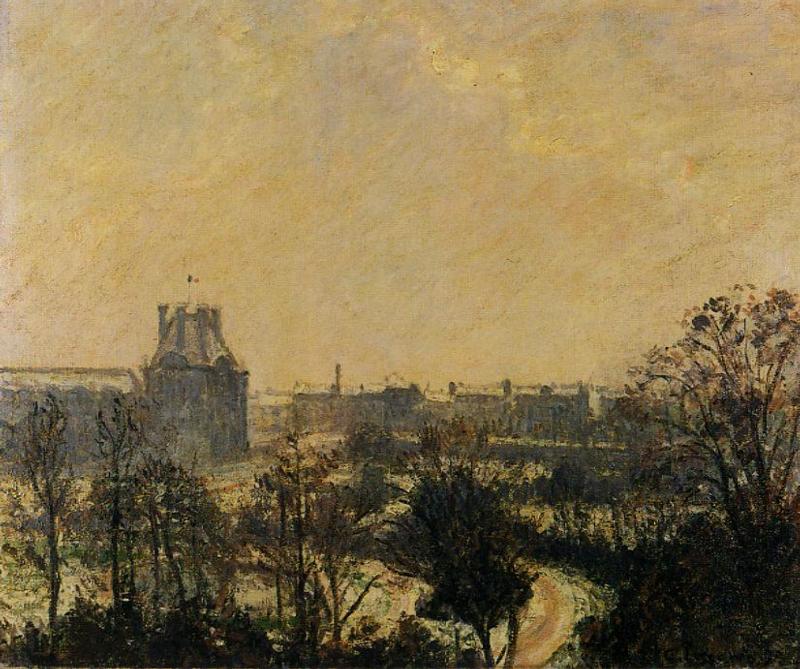The artwork, created on an off-white or antiquated paper, showcases a detailed outdoor scene with a dominant sky rendered in muted yellows, light blues, and grays. This sky, possibly done with watercolor or pastel-like mediums, appears glowing and dusky, giving a sense of an early evening or cloudy day. The foreground features dark, nearly leafless trees, depicted as silhouettes, with sparse leaves adding a touch of life. These trees contrast sharply with the bright, expansive sky. Central to the image, a pathway seems to lead into a lush area with various forms of vegetation, suggesting entry into a park or forest. Moving towards the background, the silhouette of a long line of buildings emerges, marked by a tall structure with a distinctive banner or pole. The architecture is rendered in various shades of gray, with some buildings appearing blurred and indistinct. Smudges on the lower part of the image hint at roadways or pathways, tying together the scene's natural and urban elements.